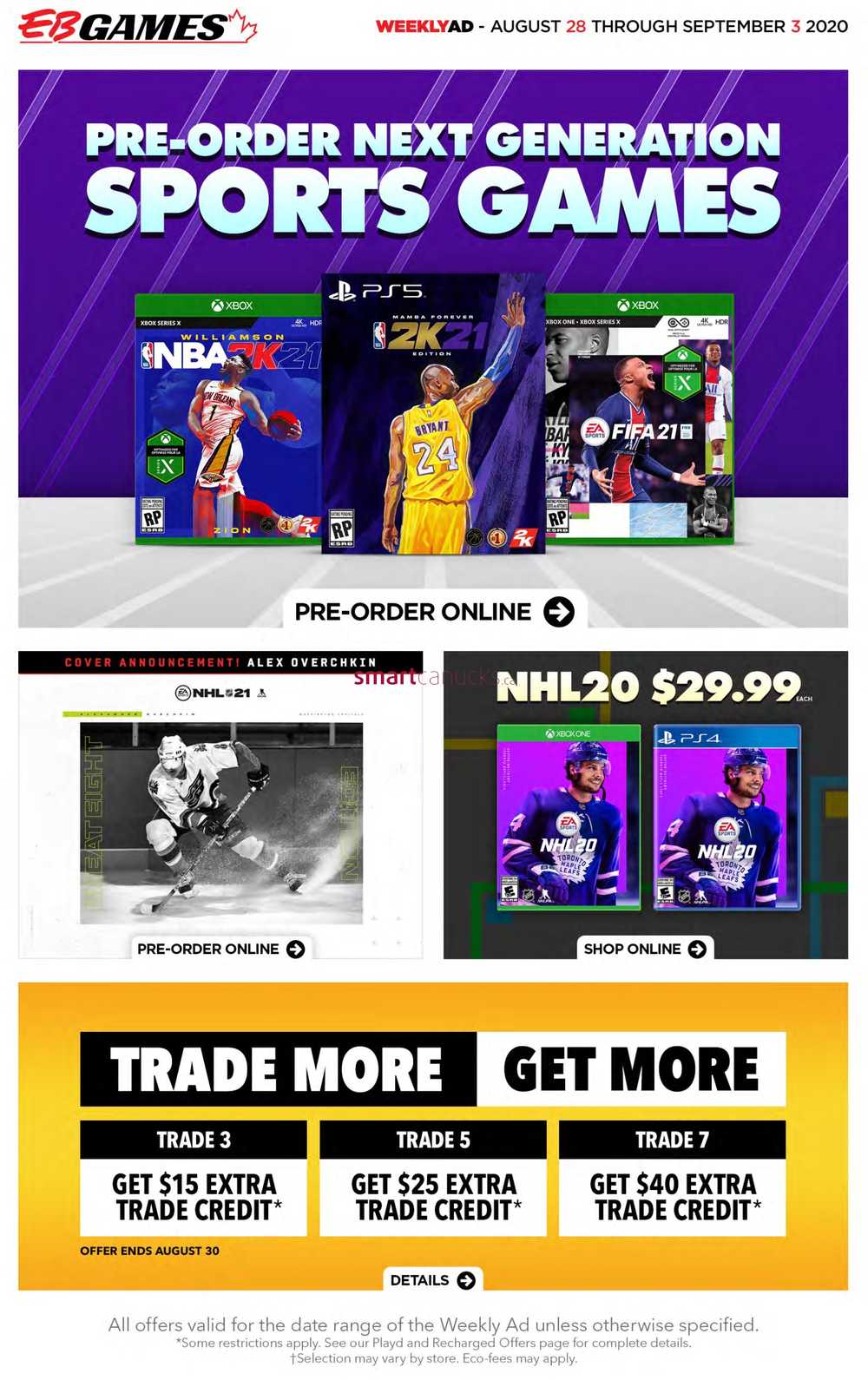This is a weekly advertisement for EB Games, a Canadian gaming retailer. At the top of the ad, there's a distinctive logo featuring a maple leaf, signifying its Canadian origin. Just underneath, in bold text, it reads "Weekly Ad, August 29th through September 3rd, 2020."

Dominating the left section of the ad is a prominent banner with the headline "Pre-Order Next Generation Sports Games." Featured below the header are three spotlighted video games available for pre-order. From right to left, we have:

1. **NBA 2K21** for Xbox, showcasing the cover athlete Zion Williamson.
2. **NBA 2K21** for PlayStation 5, similarly displayed with Zion Williamson.
3. **FIFA 21**, identified plainly without a platform specification.

Beneath these exciting game titles, the banner encourages customers to "Pre-Order Online" for guaranteed early access to these eagerly anticipated sports games. The layout and vivid imagery draw attention to the latest offerings and invite gamers to secure their copies ahead of the official release dates.